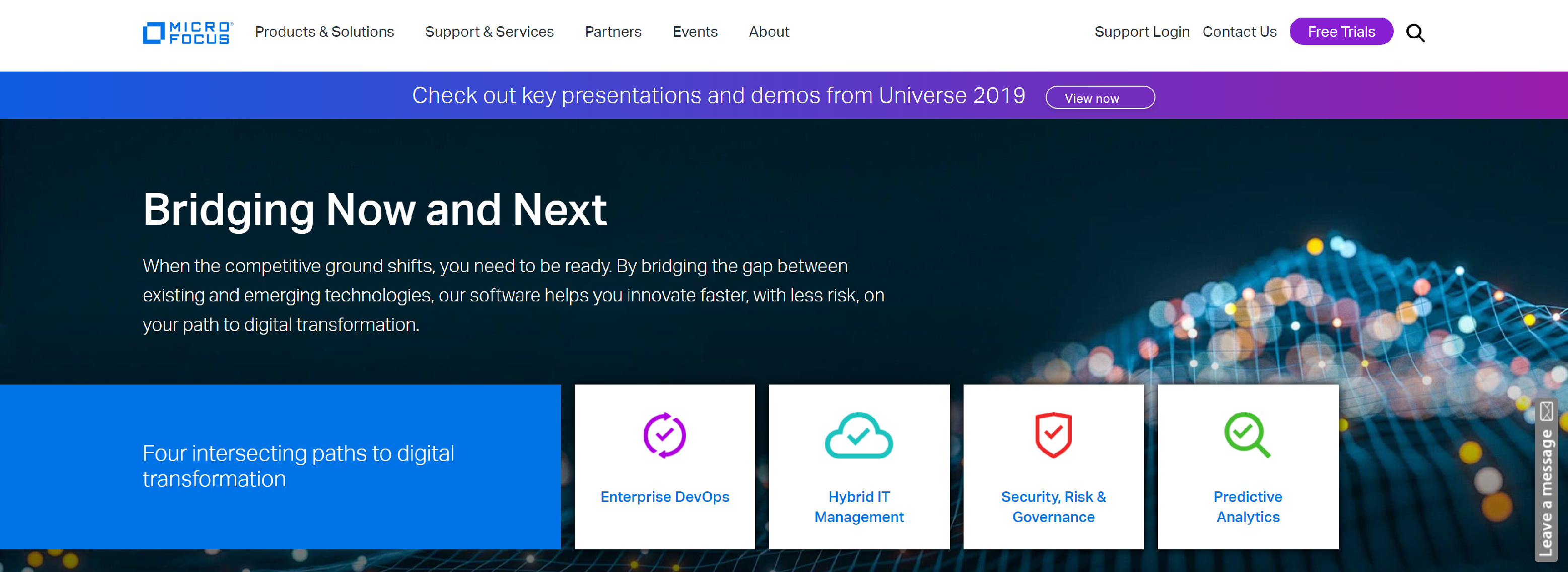The image displays the front page of a website, characterized by a sleek and professional design. At the top, the navigation bar is white, featuring the company logo on the upper left corner. The logo comprises a blue square and the company name "MICRO FOCUS" in capital letters, with "MICRO" stacked above "FOCUS". 

To the right of the logo, there are several black text subsections: "Products and Solutions," "Support and Services," "Partners," "Events," and "About." Further along, there are options for "Support," "Login," and "Contact Us," alongside a prominent pink button labeled "Free Trials" in white text. This section concludes with a black magnifying glass icon.

Below the navigation bar, a gradient banner transitions from blue to purple, displaying white text that reads, "Check out key presentations and demos from Universe 2019." A "View Now" button is situated to the right.

Further down, the main content section is set against a black background. Central to this section is the white text message: "Bridging Now and Next. When the competitive ground shifts, you need to be ready. By bridging the gap between existing and emerging technologies, our software helps you innovate faster with less risk on your path to digital transformation." 

The background imagery on the far right depicts illuminated circular lights suggesting a sophisticated network or panel setup.

In the bottom-left corner, a blue box with white text reads "Four Intersection Paths to Digital Transformation," followed by four white boxes listing transformational paths. The first box shows a pink checkmark surrounded by pink arrows and is labeled "Enterprise DevOps" in blue text. The second features a green cloud with a green checkmark, labeled "Hybrid IT Management." The third box illustrates an orange shield with an orange checkmark, described as "Security Risks and Governance." The fourth box contains a green magnifying glass with a green checkmark, titled "Predictive Analysis."

At the bottom right, a gray vertical box with white text invites users to "Leave a Message".